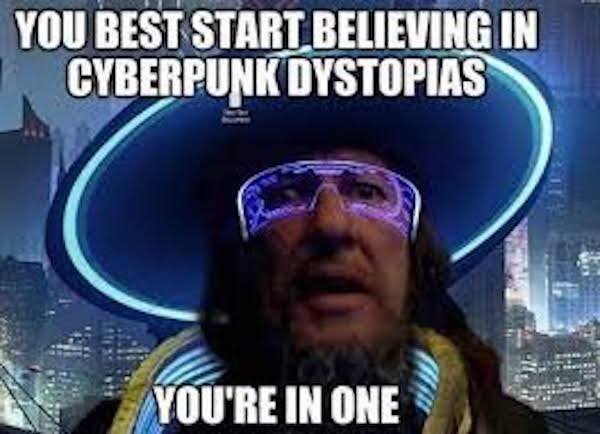In this meme-inspired image, a man stands center stage with an expression of shock or disbelief, his mouth half open. He sports futuristic 3D or VR glasses that emit a purple hue, while his head is adorned with a halo-like blue neon-lit hat extending from ear to ear. His long hair and short beard add to his striking appearance. Adding to his cyberpunk vibe, he dons a furry collar and a suit jacket interwoven with glowing light blue rods. The background is a dark, gloomy cityscape filled with tall, illuminated high-rise buildings, reinforcing the cyberpunk aesthetic. At the top of the image, bold white capitalized text reads, “You best start believing in cyberpunk dystopias,” followed by a matching text at the bottom, “You're in one.”